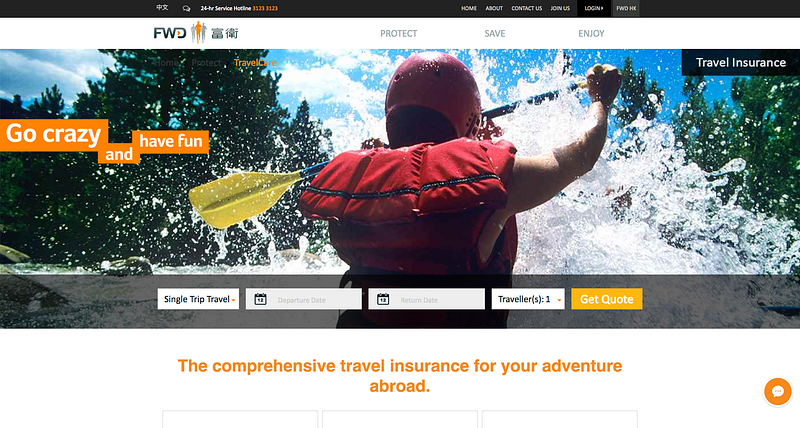**Website Screenshot Description:**

This screenshot captures the landscape mode of a website. At the top, there is a prominent black navigation bar extending from the upper left to the upper right, though its text is mostly unreadable. However, the upper right section features visible menu options labeled "Home," "About," "Contact Us," "Join Us," and "Log In."

Beneath the black stripe, a white stripe prominently displays the site's logo "FWD" followed by the tagline "Protect, Save, Enjoy" in gray text, which is somewhat challenging to read against the background.

The main visual focus of the website is a large, striking photograph of a person kayaking. The person is seen from behind, creating an immersive perspective as if we are part of the scene. The kayaker, donned in a red helmet and red protective gear, is holding a yellow oar pointed towards the left. The day is bright and clear with blue skies and scattered white clouds. The scene is dynamic, featuring turbulent white water from rapids and lush trees lining both sides.

In the upper right-hand corner, a noticeable button for "Travel Insurance" is present. On the left side of the image, the phrase "Go Crazy and Have Fun" is written in bold orange text.

Below the featured photograph, there is a form titled "Single Trip Travel." This form includes fields for entering the departure date, return date, and the number of travelers. An orange button labeled "Get Quote" follows these fields. The form is concluded with the text, "Comprehensive travel insurance for your adventure abroad."